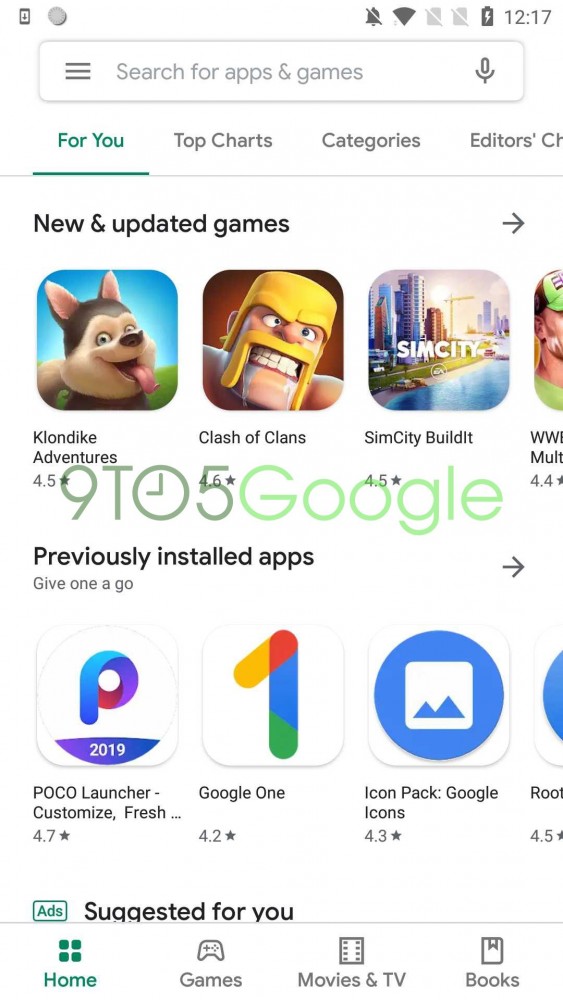This detailed screenshot captured from a tablet or smartphone showcases the user interface of an app store, likely the Google Play Store. 

On the upper left-hand side of the screen, there is an icon of a smartphone with an arrow inside, indicating an available update. Adjacent to it is a dark grey circle followed by a notification icon with a line through it, signifying that notifications are muted. Further right, a full Wi-Fi symbol indicates a strong internet connection, and two greyed-out SD card symbols with white lines through them show no SD cards are currently inserted. 

On the upper right-hand side, a battery icon with a lightning bolt indicates charging status, and the time reads 12:17, possibly in military format since it lacks an AM or PM indicator. Below, a search bar with the placeholder text "Search for apps and games" is flanked by a settings icon (three horizontal black lines) on the left and a microphone icon for voice search on the right.

The screen is bordered by a light grey rectangle housing four labeled tabs at the top: "For You," "Top Charts," "Categories," and "Editor's Choice," the latter partly cut off. The "For You" tab is selected, highlighted in green with a dark green arrow underneath.

In the main content area, under the section "News and Updated Games," there is an image of a white and grey dog and an individual in a yellow mask, followed by an icon for SimCity and another partially cut-off item. Below, "9T" with a clock face icon, and "5 Google" in light green, track recently updated apps. Further down, under "Previously Installed Apps," a suggestion reads "Give one a go" in grey.

Applications such as Poco Launcher, Google One, Drive (depicted with Google's traditional yellow, orange, red, blue, and green colors), a general icon pack, and Google Icons (a blue circle with a mountain range inside a square) are listed. 

At the bottom, "Suggested for you" is boldly highlighted, coupled with an "Ads" label in a green rectangular box on the left. The navigation bar at the very bottom shows "Home" (indicated by four green squares and is selected), "Games" (depicted with a controller icon), "Movies and TV" (indicated by an old movie reel icon), and "Books" (represented by a square with a bookmark symbol), in grey.